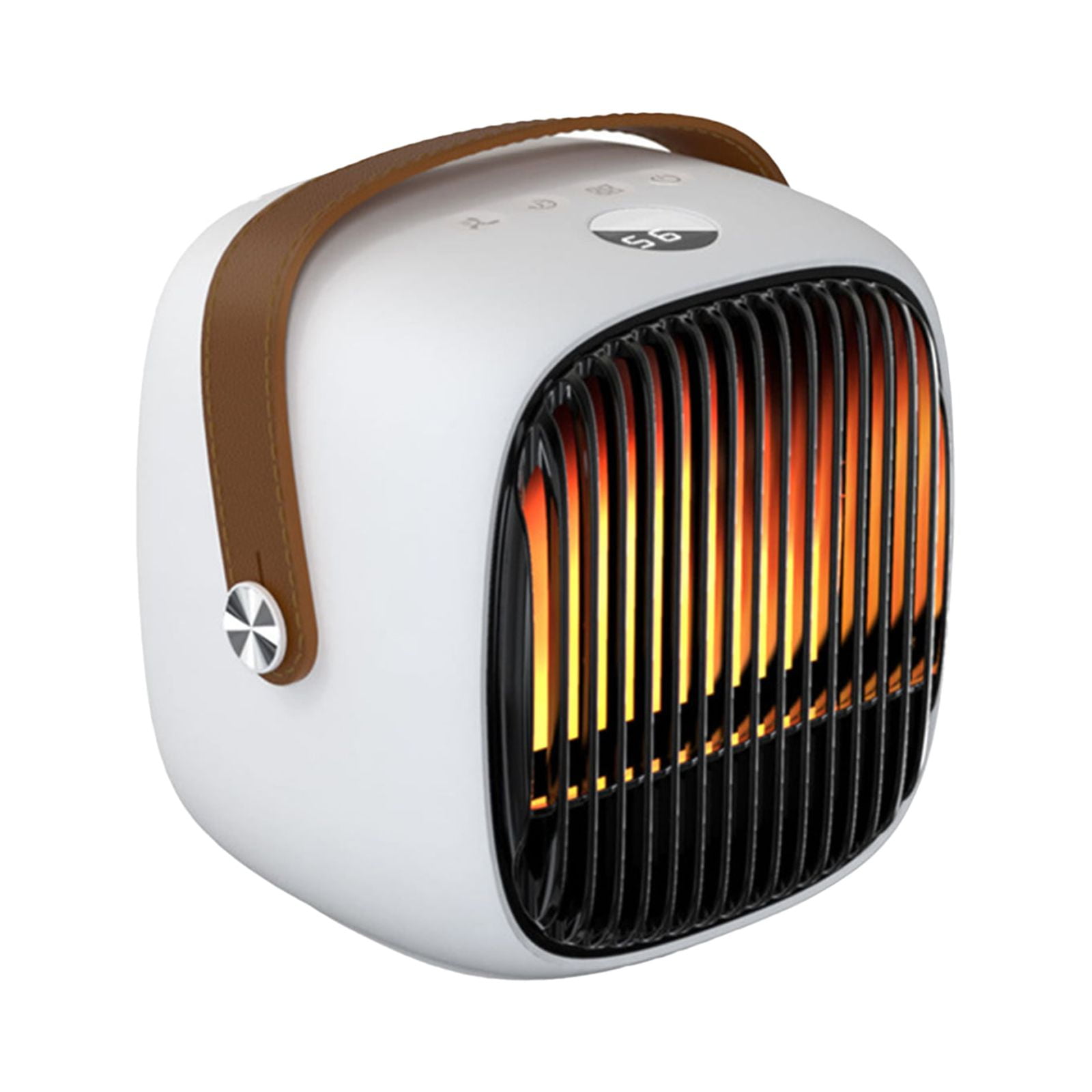This image is a detailed, angled stock photo of a compact, cube-shaped portable heater with rounded edges. The heater is predominantly white, constructed from hard plastic, and features a distinctive brown leather handle attached to the top, capable of spinning from left to right for easy carrying. A round plastic piece with a silver front secures the handle to the device. Prominently displayed at the top of the heater is a round silver circle displaying the temperature, as well as a row of four small buttons and one larger button that is white and black with the number "56" on it. 

The front of the heater is black and grated, showcasing a vivid orange glow from the heat source within. The heater’s grill consists of vertical black lines, through which the yellow, orange, and red hues of the glowing light can be seen. The device is set against a transparent background, emphasizing its clean and modern design. The heater's grates are oriented to the right, highlighting its angled presentation in the image.